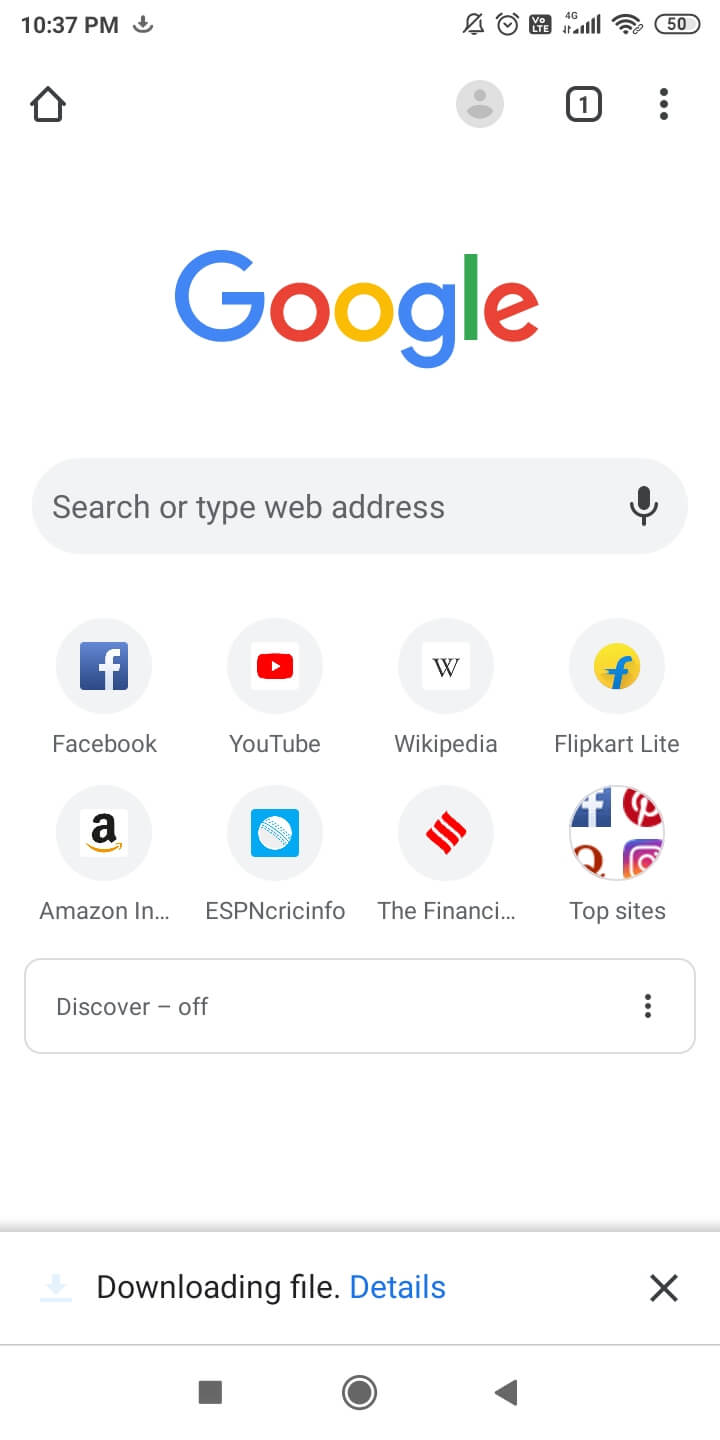A screenshot of a mobile device captured at 10:37 PM. In the top right corner, various icons are displayed alongside a battery indicator showing 50% health. The screenshot features the Google homepage viewed in the Chrome browser, distinguishable by its Chrome UI elements. The screen prominently showcases the classic Google logo with the search bar beneath it. Below the search bar, there are thumbnails of recently visited websites, including Facebook, YouTube, Wikipedia, Flipkart Lite, Amazon, ESPN, Cricinfo, and the Financial Times, among other top sites. Toward the middle of the screen, a section titled 'Discover’ appears, which has been turned off, leaving a noticeable white space. Below that, there is a notification stating 'Downloading file' with a blue 'Details' link that can be dismissed by an 'X' button. At the very bottom of the screen, there are three navigation buttons: a square (Recent Apps), a circle (Home), and a triangle (Back), all shaded in a darker gray color.